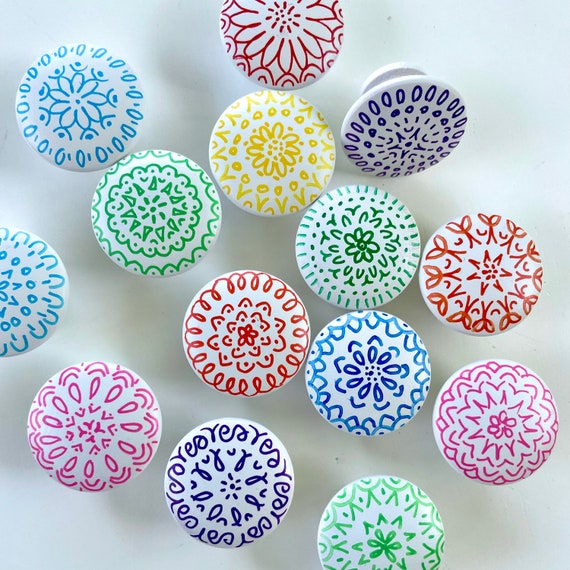The image features a light gray background adorned with an assortment of large, decorative buttons, each showcasing unique and colorful floral designs. Among the collection, there are prominent red buttons adorned with bold red flowers. Additionally, there are white buttons embellished with flowers in various colors: blue, green, yellow, purple, light orchid, light green, very light purple, and pink. Each button is meticulously detailed with intricate floral patterns, enhancing their visual appeal. One button is displayed sideways, revealing its back and illustrating the mechanism where the button passes through a single hole, while the decorative face remains visible on the exterior.